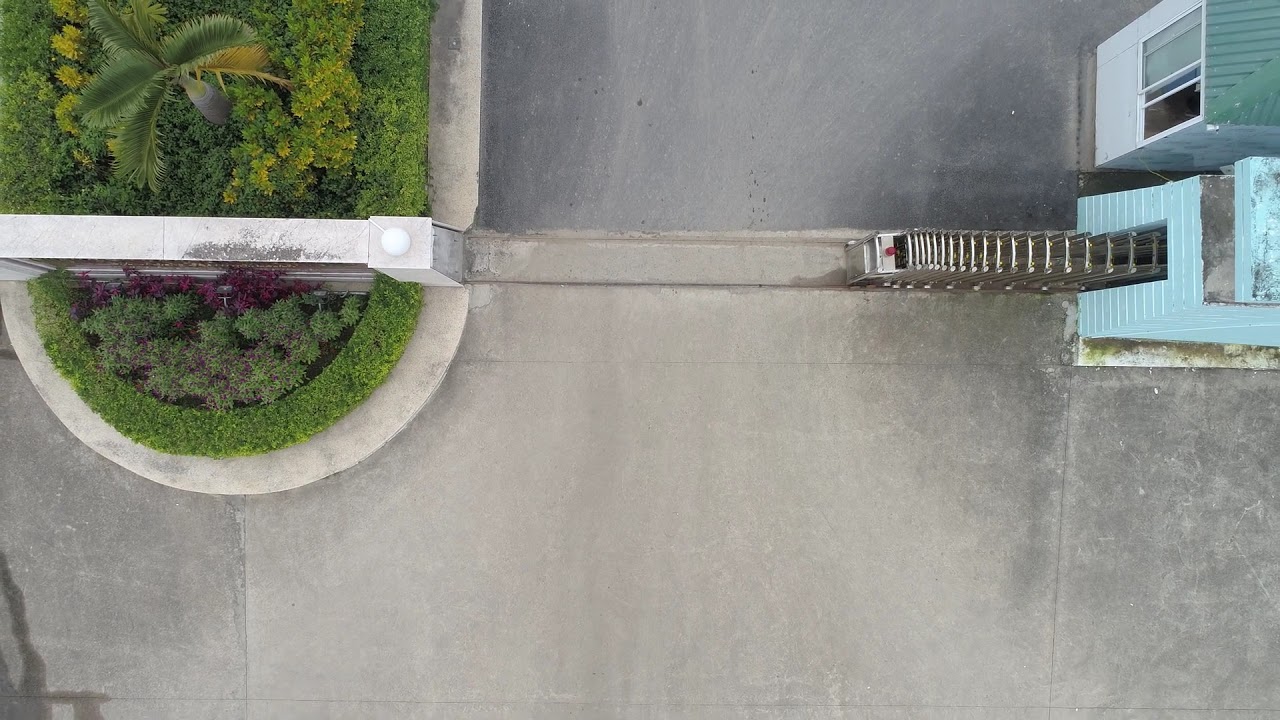This overhead view captures a paved area, approximately 35-40 feet below, showcasing a cement expanse that dominates the image. To the upper left, there's a landscaped section featuring green vegetation, including bushes and possibly a palm tree, bordered by circular concrete edging. Extending through part of this landscaped area is a white-topped wall, punctuated by a column with a round, likely illuminated, fixture atop it.

The dominant feature on the right side of the image is a row of shopping carts, neatly lined up, suggesting they are positioned for easy access outside an adjacent structure. This structure, painted in a light blue hue, appears to be part of a larger building, possibly a store, as inferred from the shopping carts characteristic of retail establishments. Above this is another structure with windows, further anchoring the scene in an urban or commercial setting.

Despite the lack of people, text, or vehicles, the image is rich in color variations, featuring shades of aqua, light aqua, white, green, yellow, and gray. This detailed composition outlines a functional outdoor space linked by pathways and bordered by a mix of natural and built elements, hinting at a commercial or gated community entrance.